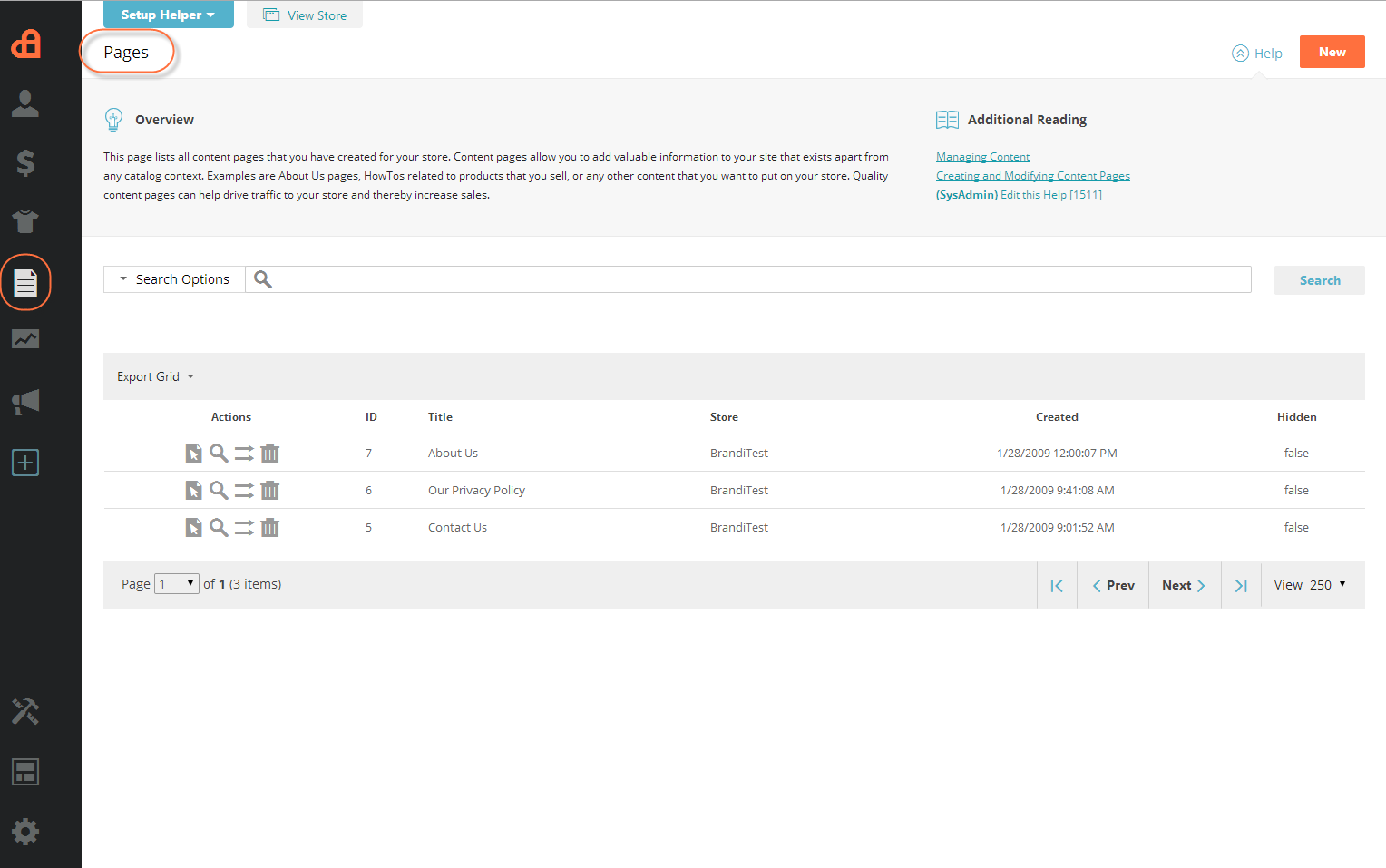This image depicts a webpage interface, likely part of a website's content management or administrative panel. Dominating the upper area of the interface, the word "Pages" is prominently displayed and circled in orange. Just above this, there are two distinct boxes: a blue one labeled "Setup Helper" and a white one saying "View Store."

Down the left side of the screen, there's a vertical black sidebar containing various icons. The first icon appears to be heart-shaped, and notably, there is a letter-shaped icon circled in red among them.

To the right, the webpage is divided into multiple sections. In a gray-shaded area titled "Overview," you can find a subheading labeled "Additional Reading." The "Additional Reading" section features blue-colored, clickable text links for further information.

Centrally located on the page is a search section marked by the title "Search and Options." This includes a search bar with unreadable, drop-down content beneath it that offers further functionalities or settings. Midway through the page, there is some content that is not clearly discernible. At the bottom, it states "Page 1 of 1," indicating that this is the sole page currently being viewed.

In the upper-right corner of the interface, there is an orange box labeled "New" next to a blue "Help" link, providing additional assistance options for the user.